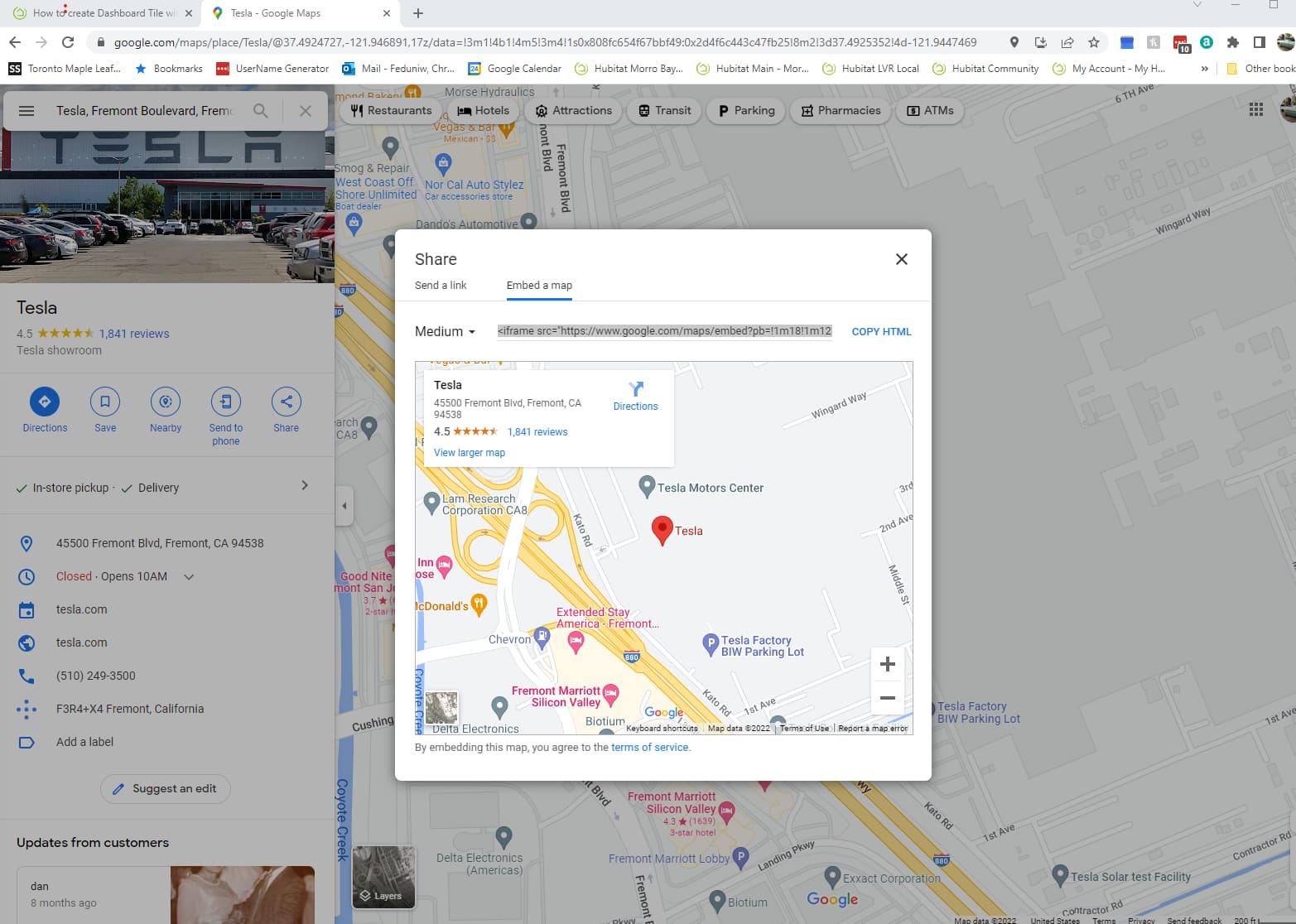Displayed is a detailed screenshot of a Google Maps interface with various elements and tabs. In the top left corner, there is a grayed-out tab titled "Create Dashboard Title," indicating it is not currently selected. Adjacent to it is a selected tab labeled "Tesla," under which "Google Maps" is displayed.

Below the top bezel, which is white, there is a black arrow pointing to the left, and a grayed-out, non-functional gray arrow pointing to the right. There is also a black refresh symbol present. The URL bar shows an exceptionally long web address.

Further down are multiple tabs, each with distinct icons and partial labels:
- A tab with a black square featuring white "SS" initials, labeled "Toronto Maple Leafs," but truncated with ellipses.
- A bookmarks tab marked by a blue star.
- A red square with white ellipses, labeled "Username Generator."
- A blue square with another darker blue square overlay, labeled "Mail."
- A tab partially labeled "FEDUNIWCHR" followed by ellipses.
- A Google Calendar tab, represented by a half-blue, half-green, and half-yellow square marked with the number "24."
- Tabs labeled "Habit Morrow Bay," truncated to "Habit Morrow" and "Habit VR Local."
- Additional tabs labeled "Habit Community," "My Account," "My," followed by a dash and partially visible "My H."

On the left side of the screen, there is a visual of the Tesla location, showing several cars in front of a Tesla building. The listing displays a rating of 4 out of 5 stars based on 1,841 reviews, with the rating being clickable in bold blue text. There are various action buttons displayed as circles beneath this: a dark blue "Directions" button (indicating it is selected), along with "Save," "Nearby," "Send to Phone," and "Share" buttons. A red label indicates that the location is currently "Closed" and will open at 10 AM.

A pop-up window in the screenshot shows map sharing options. The selected option is "Embed a Map." On the left side, the option "Send a Link" is also available. At the top, "Share" is bolded in black. A black "X" in the top right corner indicates the option to close the pop-up.